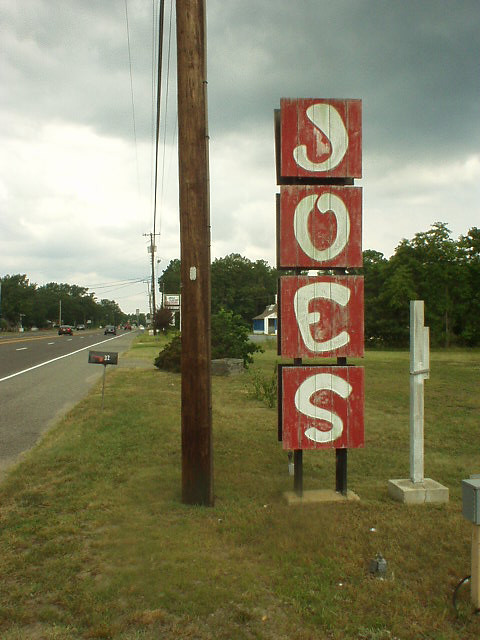This photograph, oriented as a portrait, captures a scene taken from the side of a four-lane road. The road extends from the left center of the image into the distance, marked by a solid yellow line in the middle and white dashed lines, with cars visible traveling in both directions. The foreground includes a gravel shoulder and a grassy area where the photographer seems to be standing.

Central to the image is a tall, brown wooden power line pole. Just to the right of this pole, there is a prominent sign for "Joe's." The sign consists of four vertical, square panels, each made from five wooden planks painted red with faded white hand-drawn letters spelling out J-O-E-S from top to bottom. These panels show significant weathering, revealing some raw wood beneath the chipped paint.

The sign appears to be mounted on a dual post structure and is echoed by equally sized panels on the opposite side, making it visible from both directions. There's also mention of a small, illegible sign next to it and a black mailbox down the road. Beyond the sign and pole, the background is filled with plenty of green trees under a grey, gloomy sky, adding a somber tone to the photograph.